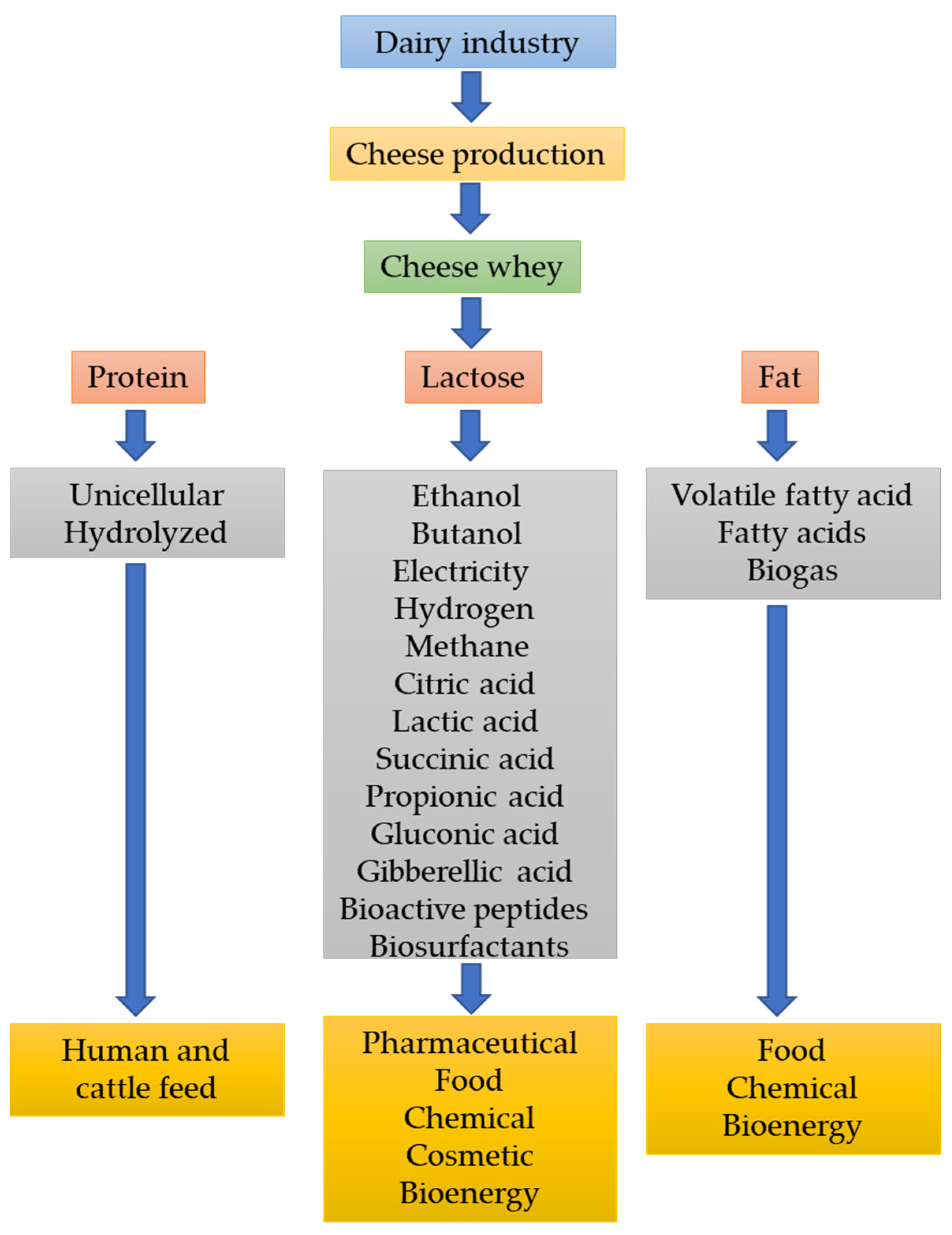This detailed diagram illustrates the flow of processes within the dairy industry using colorful bubbles and arrows. At the top, the chart begins with the dairy industry, leading to cheese production, which then results in cheese whey. The whey is divided into three categories: protein, lactose, and fat. 

The protein branch indicates a sequence towards unicellular hydrolyzed substances, which ultimately serve as human and cattle feed. 

The lactose pathway, shown in a central column, highlights its derivatives: ethanol, butanol, various acids (citric, lactic, succinic, propionic, gluconic, gibberellic), bioactive peptides, and biosurfactants. This pathway culminates in applications across several industries, including pharmaceuticals, food, chemicals, cosmetics, and bioenergy. 

On the right, the fat category transitions to volatile fatty acids, fatty acids, and biogas, which are further utilized in food, chemical, and bioenergy sectors.

The diagram uses a variety of colors—blue, red, gray, green, yellow, and gold—to distinguish different sections, making it a vivid representation of how raw dairy product components are transformed into a wide range of commercial and industrial products.